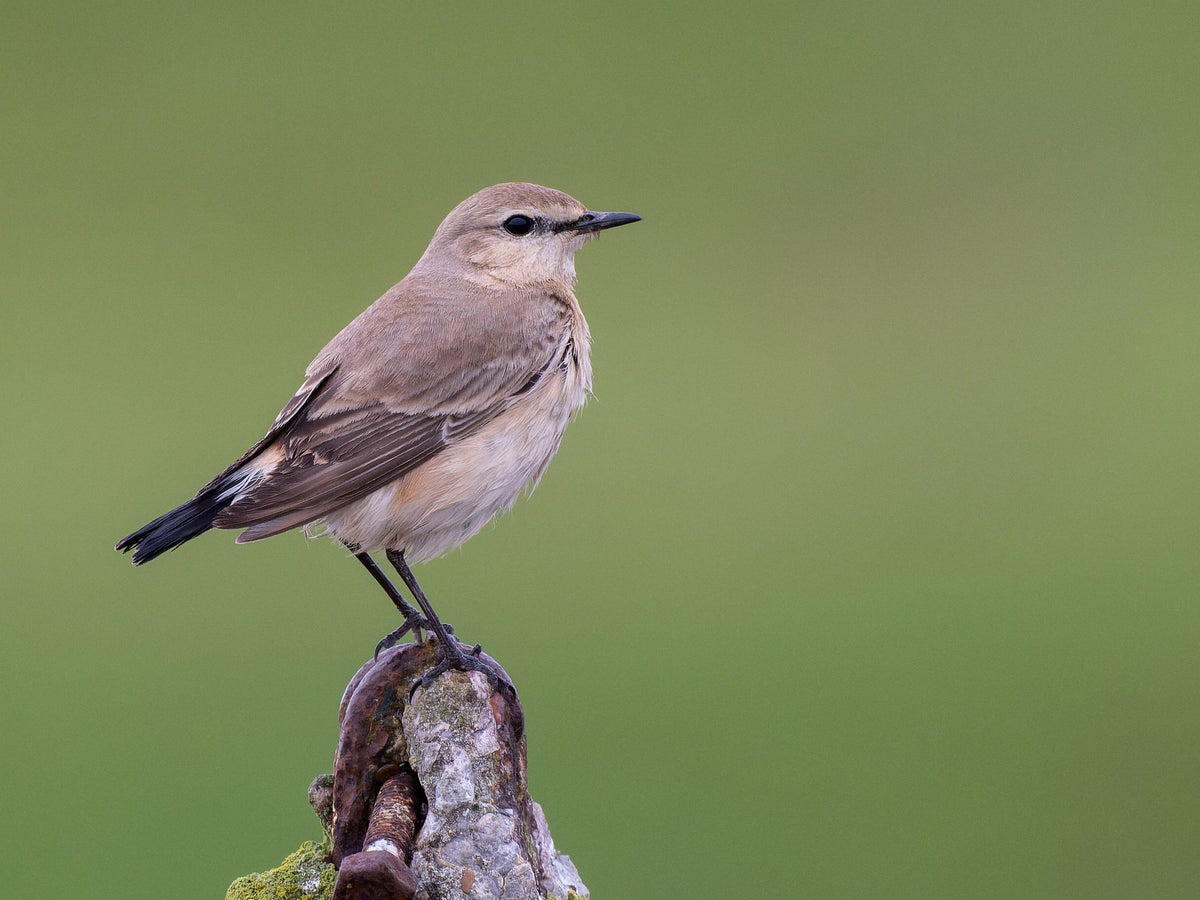This detailed image features a very small bird perched on a rusted piece of metal equipment, positioned towards the left side of the frame. The bird is primarily grayish-brown with subtle shades of tan and gray on its back and head. Its underbelly is a soft gray, accented with a hint of peach near its legs. Distinctive markings include black tail feathers, black wing tips, and a sharply pointed black beak. The bird's legs and eye are also black, adding to its intricate appearance. The rusted metal it perches on is weathered, displaying a mix of light gray textures and rusty red patches with a large rusted bolt visible at the top. The blurred background features a greenish-gray hue, reminiscent of natural foliage, creating a serene and aesthetically pleasing environment around the bird.